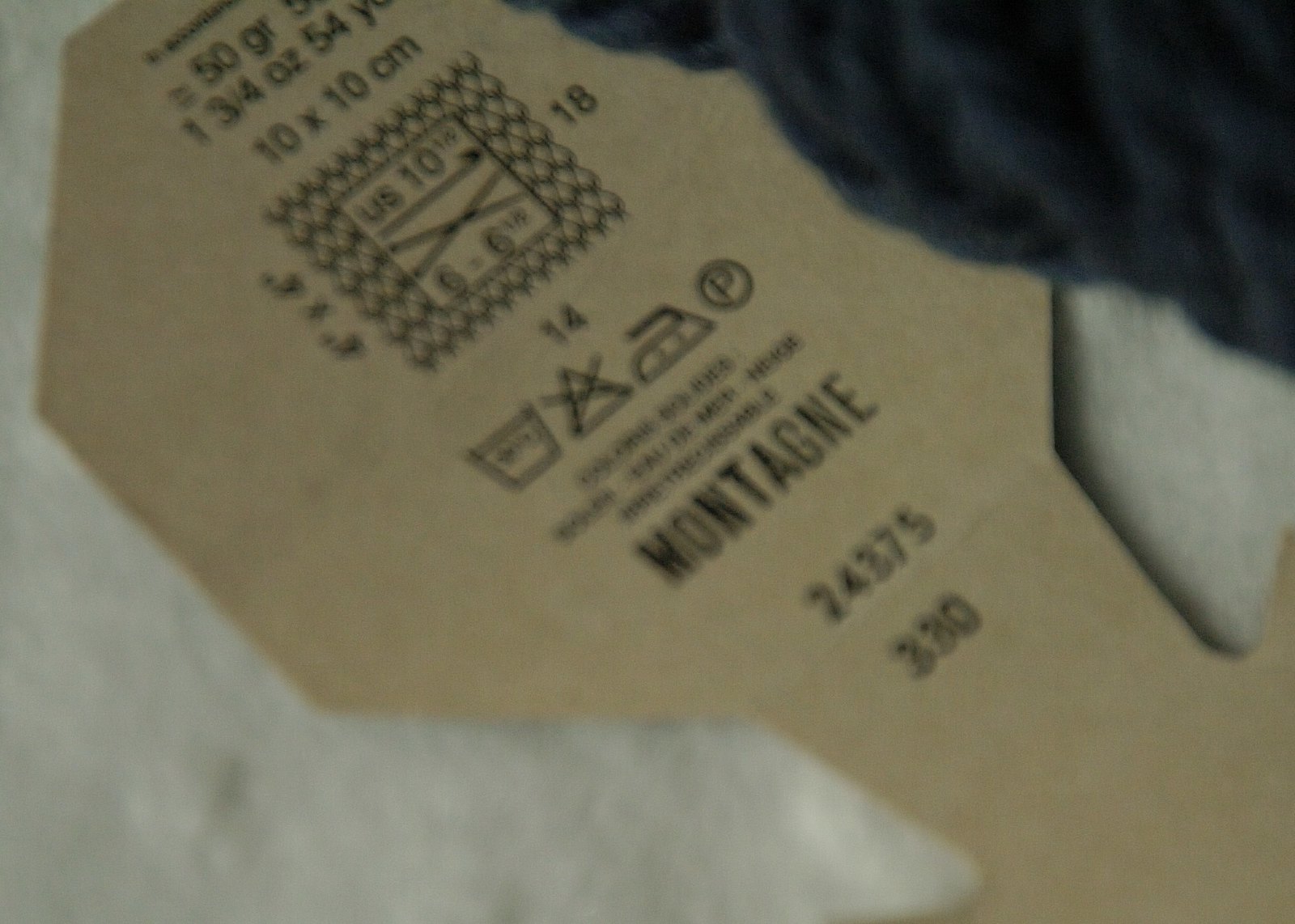This image features a blurry close-up of a tag, with the prominent text "Montague" displayed. The tag appears to have European origins, as indicated by measurements provided in both grams and ounces: "50 grams" and "1 3/4 oz." Although the precise purpose of the tag remains unclear, it likely belongs to a piece of clothing or fabric, given the presence of weight measurements and an icon suggesting it can be ironed. The tag is placed against a white background, accompanied by a fabric piece that is either blue or gray in color. Unfortunately, the text above "Montague" is illegible due to the blurriness of the image, adding an element of mystery to the tag's complete information.